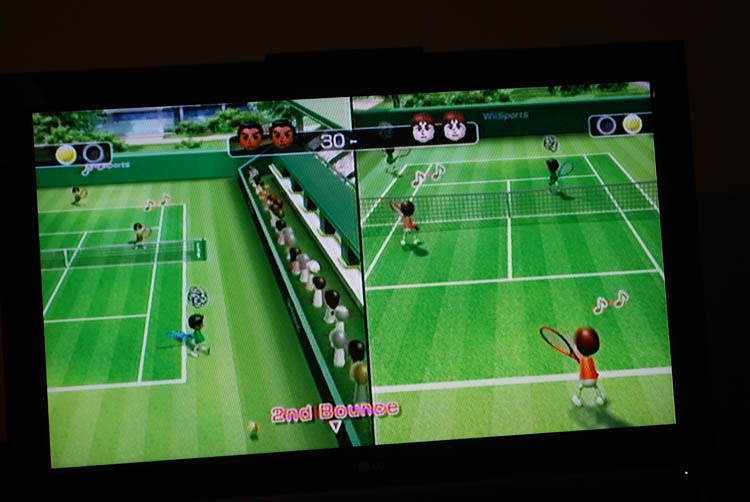In this image, we see a photograph of a screen displaying the video game Wii Sports Tennis in split-screen mode. Each half of the screen shows different angles of a vibrant, green grass tennis court with white boundary lines and a visible net dividing the court. One side features two avatars dressed in red shirts, and the other side features two avatars in green shirts. Both sides of the net have player avatars; on the closer side, the dark-skinned avatars are playing against light-skinned avatars positioned further away, some of whom have musical notes above their heads, indicating some form of status effect in the game. The top of the screen shows game-related information, including the score, player names, and the number of balls, while the bottom displays "Second Bounce" in red text. Background details include a house, bushes, audience members in the stands, and the overall screen is captured slightly askew with everything outside it engulfed in darkness.